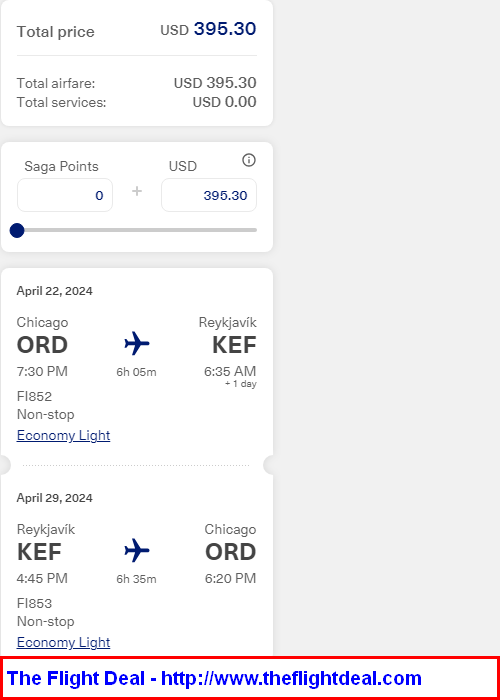A cropped screenshot of flight information highlights the pricing details at the top. The total price is prominently displayed in blue as $395.30, broken down into total airfare and services within a white box. Beneath this, a smaller white box notes "Saga points" set to zero, alongside the cost in US dollars. A movable bar adjusts Saga points, but it's currently set to zero.

Further down, the screenshot resembles a ticket, detailing departure and return information. It shows the departure date, airport codes, and corresponding flight details. The second portion of the ticket outlines the return on April 29, 2024, listing the departure and destination airports.

At the bottom of the screenshot, there is a link to theflightdeal.com, emphasized with a red box, indicating this flight deal originates from that site.